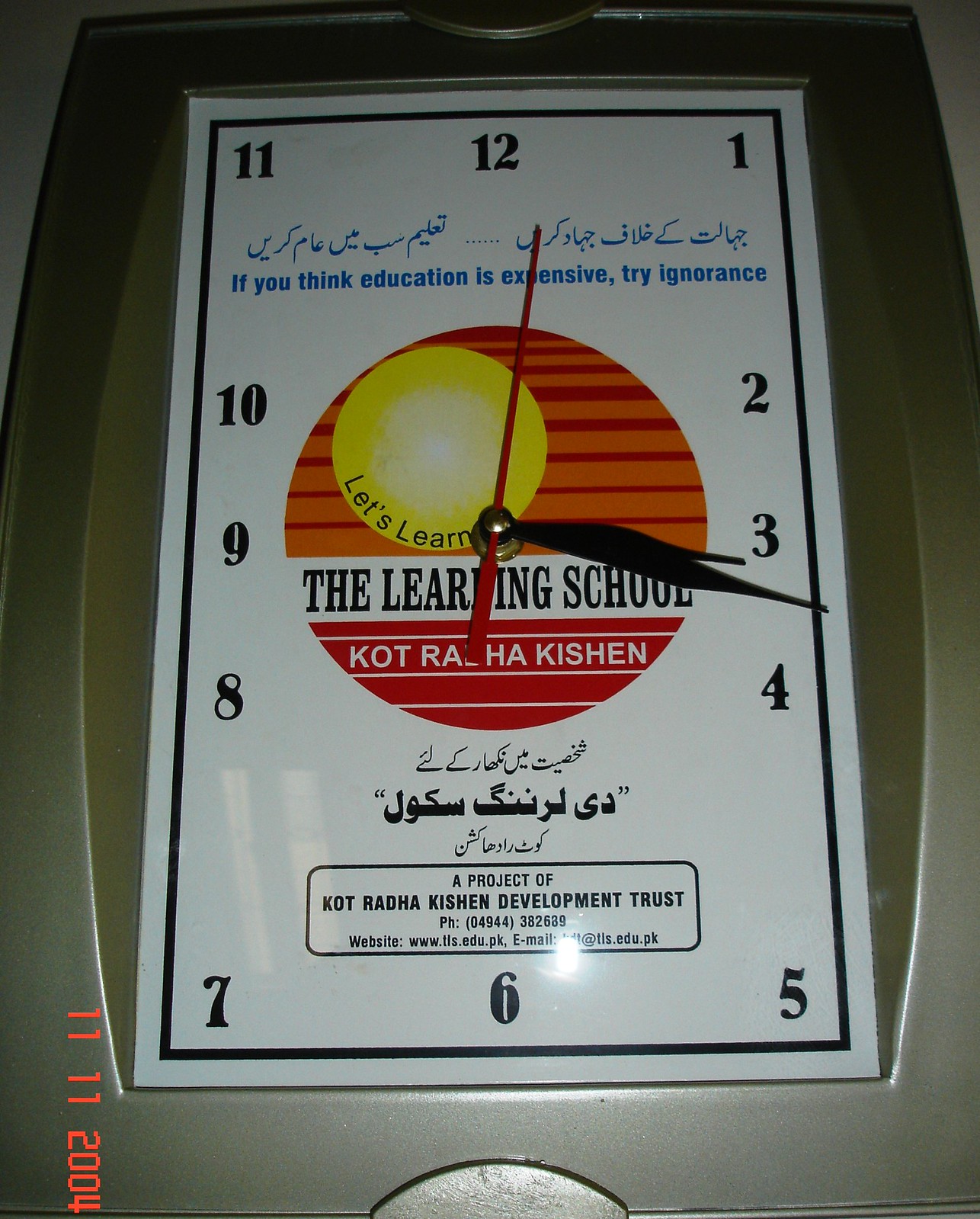**Caption:**

This image features a uniquely handmade clock, possibly crafted on a cardboard or similar material. The clock functions as a timetable, indicating opening hours. The background is predominantly white with a subtle inset black border. At the top of the clock is the 12 o'clock mark, with hours arranged sequentially around the face, mimicking a traditional clock layout.

At the center of the clock, where the hands are fixed, there is a vibrant, scaled pattern in shades of red and orange, with a bright yellow dot at the very center. The clock face prominently displays the text "Let's Learn" and "The Learning School, Katraha Makhishan." The clock hands are positioned around 3:18, while the second hand is just past the 12 o'clock mark.

Below the numbers, there is text in another language, possibly Arabic, written in blue. Additionally, the phrase "If you think education is expensive, try ignorance" is also displayed in blue text. Underneath the clock, three rows of Arabic script are evident in black. 

A small box beneath these rows contains the text "A project of Katraha Makhishan Development Trust," followed by a phone number and a website. The visibility of some details is slightly obscured due to a reflective shine on the surface. The entire arrangement is set against what appears to be a silver metal base, adding a refined touch to the overall design.